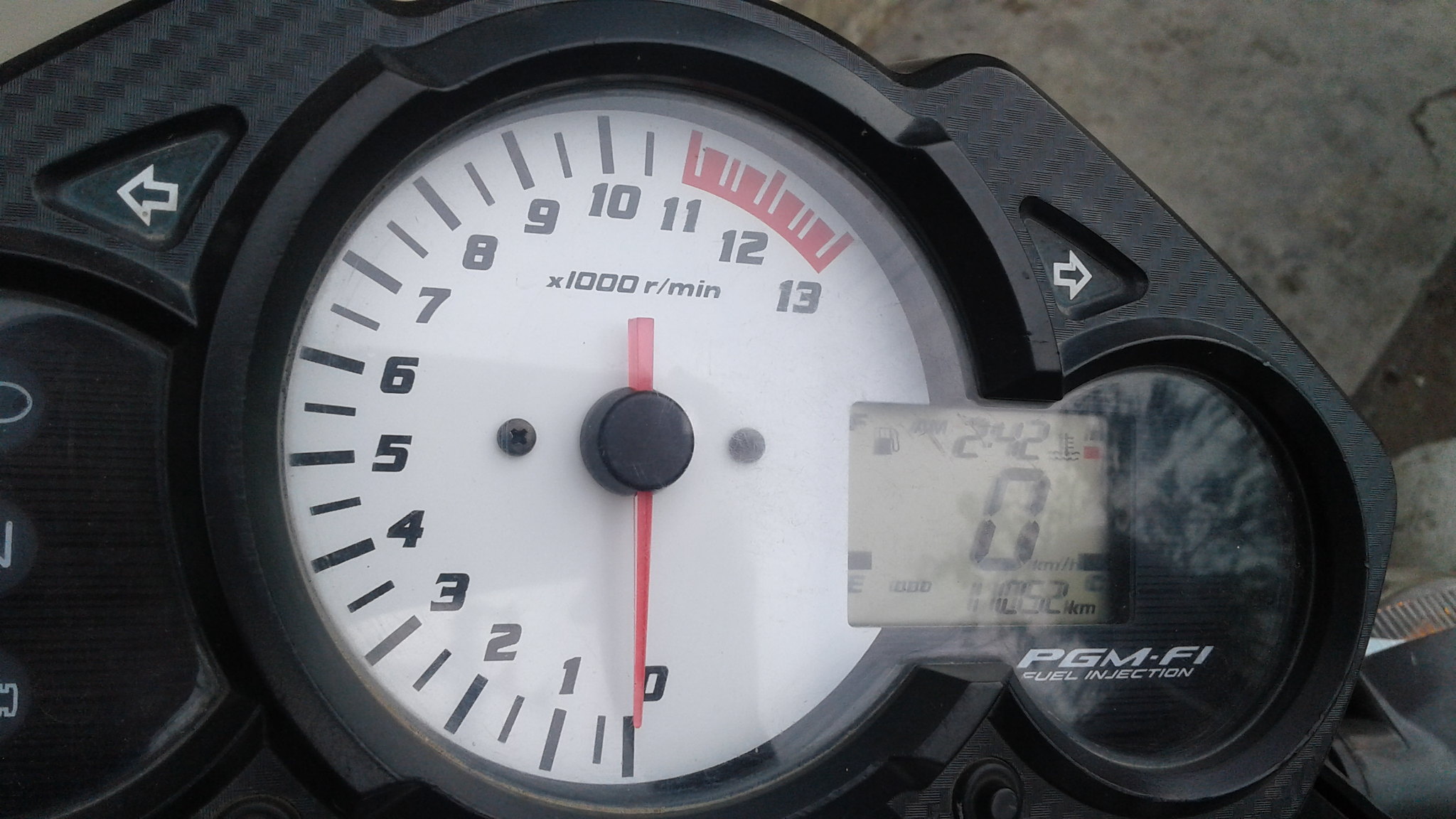The image shows a close-up view of a motorcycle's tachometer gauge, designed to measure revolutions per minute (RPM). The gauge features a circular face with a white background and is dominated by a large red needle that indicates RPM levels. The measurements start at zero at the 6 o'clock position and ascend clockwise until they reach 13 at approximately the 2 o'clock position. The right side of the gauge is blank, indicating that the scale maxes out at 13. The numbers 11, 12, and 13 are highlighted in red, signifying the redline area of the tachometer. The fine print on the gauge reads "x1000 r/min," indicating that each numerical increment represents 1000 revolutions per minute.